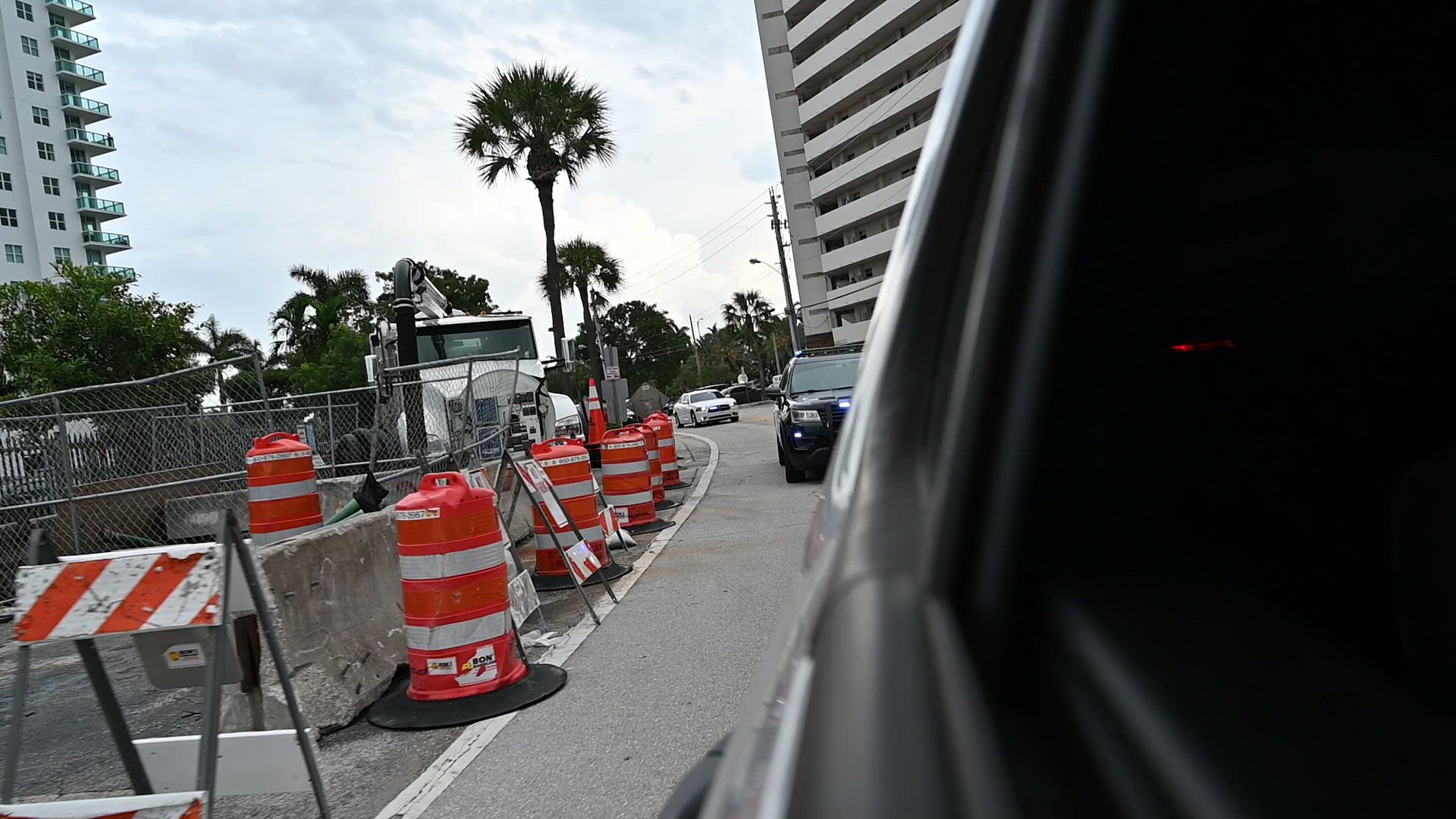This image captures a bustling downtown area of Phoenix, Arizona, under a mostly cloudy midday sky. The scene is characterized by an array of white, puffy clouds with patches of blue peeking through. A variety of palm trees, including both date palms and other species, dominate the landscape, adding a distinctive Southwestern aesthetic. The abundance of palm trees punctuates the urban setting, offering a stark yet harmonious contrast to the modern cityscape.